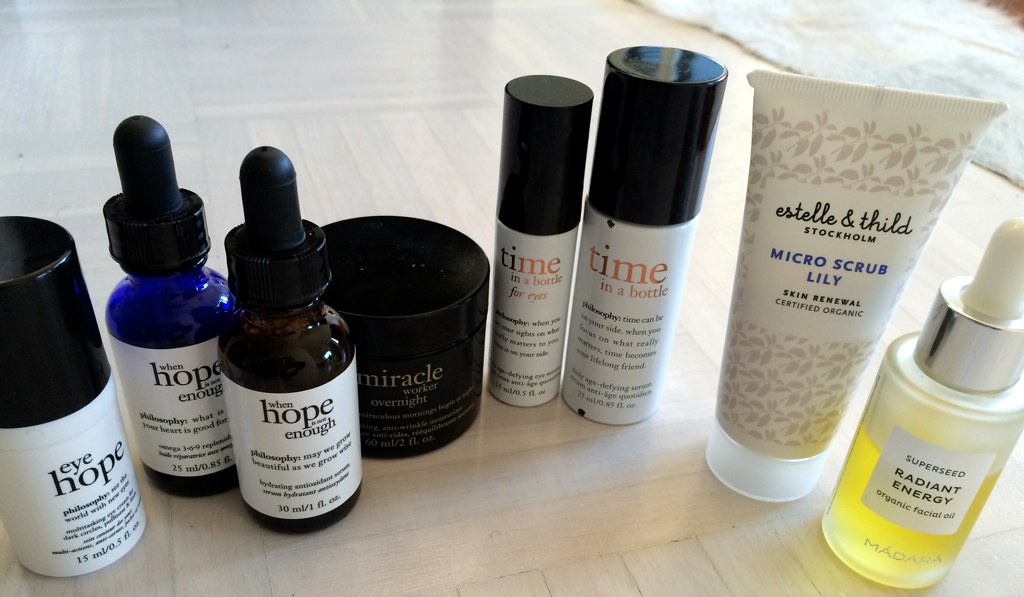The image is a meticulously arranged flat lay photograph of various beauty supplies, showcasing an array of bottles and containers.

On the far left sits a pristine white bottle with a sleek black cap, prominently labeled "I HOPE." Adjacent to it are two bottles positioned diagonally from each other, each brandishing the intriguing text "WHEN HOPE SOMETHING ENOUGH." 

Behind these, a short black candle stands out with its bold inscriptions "MIRACLE" and "MIDNIGHT." The adjacent duo consists of two taller, slimmer bottles; the left one is the more slender of the two, marked with "TIME IN A BOTTLE FOR EYES," while its counterpart to the right shares a similar design and font but simply reads "TIME IN A BOTTLE."

Further to the right, a tan bottle adorned with a distinctive pattern captures attention. It is a lotion bottle labeled "ESTHEL ENTHYLED MICRO SCRUB LILY SKIN RENEWAL." Finally, on the far right, a glass bottle with a squeeze dropper lid and a silver band catches the eye. This elegant bottle, filled with yellow liquid, is labeled "SUPERSEED RADIANT ENERGY ORGANIC FACIAL OIL."